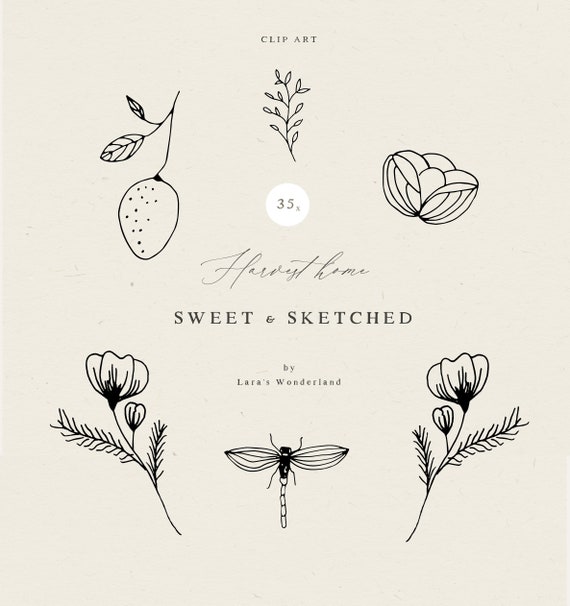This image showcases a detailed piece of clip art on a plain light gray background. At the top, the text "Clip Art" is displayed prominently. Directly below this text is an illustration of a branch with simple oval leaves, and to its left, a fruit resembling a strawberry hangs from a smaller branch. Nestled in the center of the composition, beneath the main branch, is a white circle with the number "35" inscribed within it. Below this, in elegant cursive script, the words "Harvest Home" are featured. Further down, a bolder all-capitalized font reads "Sweet and Sketched by Laura's Wonderland." Towards the bottom center of the image, a stylized dragonfly is depicted, flanked on either side by mirror-image flowers with feathery fronds instead of leaves. In the upper right-hand corner, there is a figure made of several elegant curves, resembling the top part of a flower beginning to open. This detailed compilation of black ink line art against a subtle gray backdrop reflects a harmonious blend of nature-themed elements arranged in an aesthetically pleasing manner.